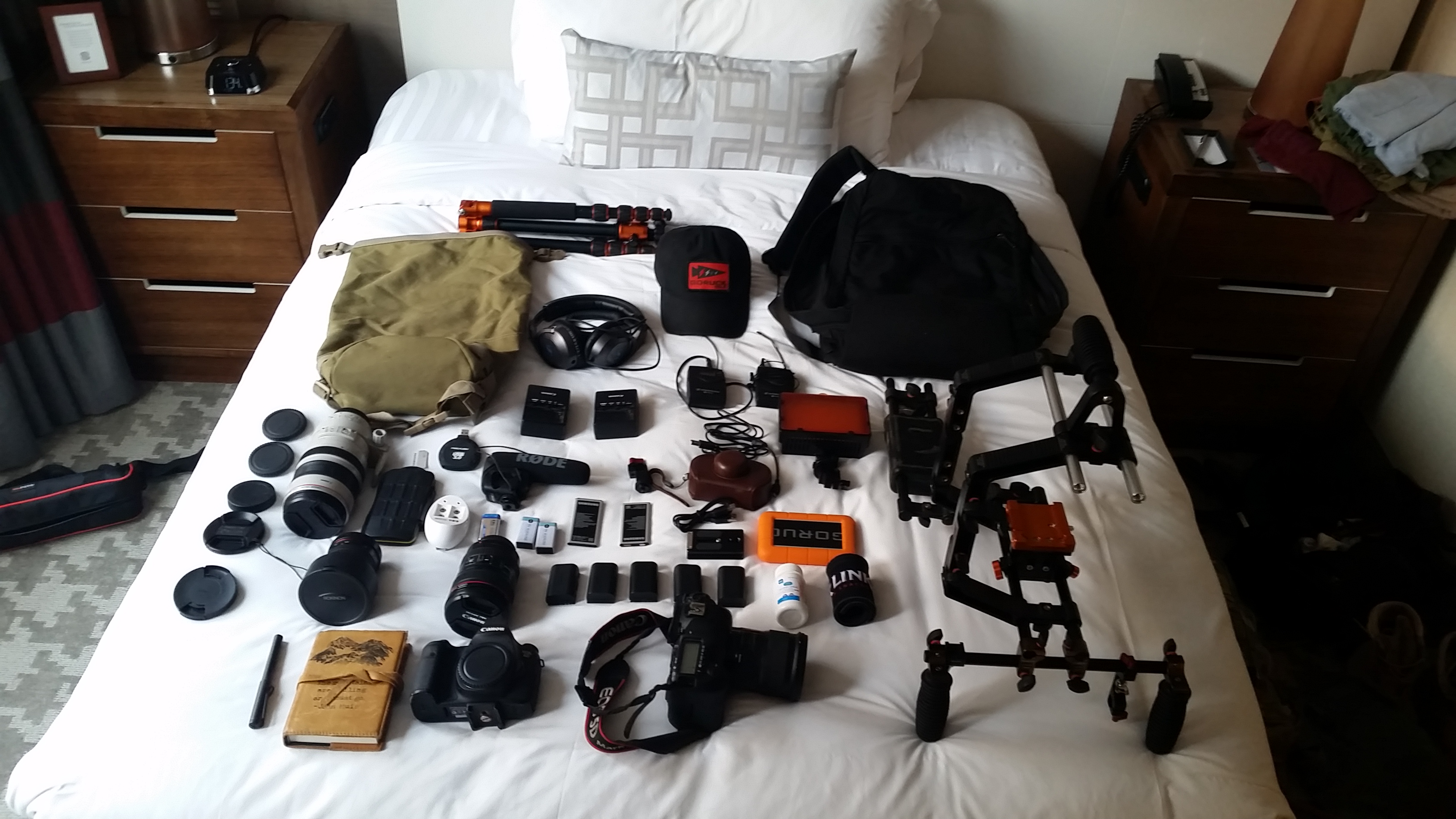In a cozy bedroom, likely a hotel room, a horizontal-rectangular image showcases a single bed neatly covered with white sheets, pillowcases, and a white comforter. Resting against the white pillows is a gray and white block pillow. Spread out meticulously across the bed is an array of camera and electronic equipment, seemingly prepared for assembly or use. Towards the bottom left of the bed, a brown checkbook and a pen lie alongside a variety of dark-colored parts. Among these parts is an orange digital timer and a strikingly large, black, round object situated closer to the pillows.

The array includes several camera lenses with their caps off, and two cameras further complement the collection. Scopes are scattered neatly, and an olive green backpack rests at the top left corner while a black backpack occupies the top right. Positioned near the center of the bed towards the top is a black baseball cap adorned with a red patch. A tripod stand and a pair of over-ear headphones are also visible.

Adjacent to the bed, twin brown nightstands anchor each side, potentially part of matching furniture in the room. The floor around the bed features a carpet in two shades of gray, enhancing the room’s soft ambiance. This detailed arrangement provides a glimpse into the methodical organization of someone meticulously preparing their equipment, possibly for an upcoming shoot or project.